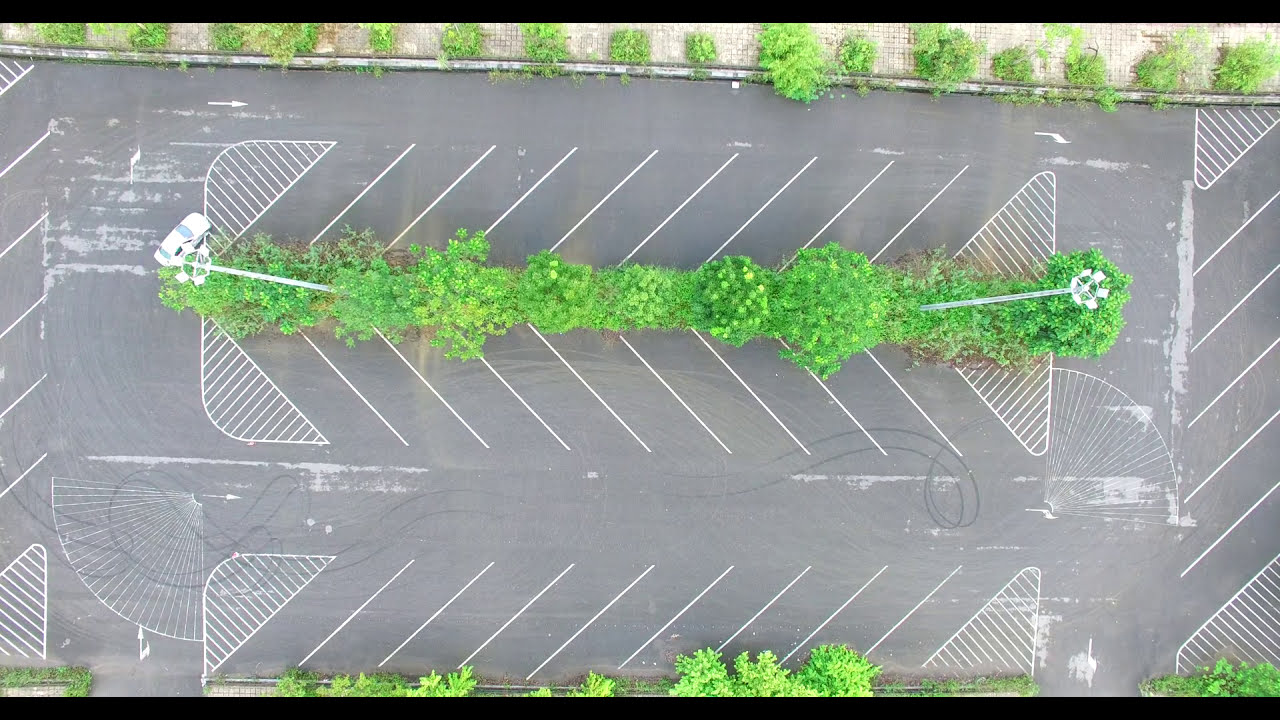The aerial image captures a concrete parking lot, characterized by a structured layout of angled parking spaces and several green median strips. The parking lot features three central rows of angled parking spaces, each containing about nine spots, and two additional rows on either end with approximately six spaces each. A distinctive green strip of bushes runs horizontally through the middle of the lot, separating the central rows. More greenery is visible at the top and bottom edges of the image, interspersed with patches of deteriorating paving. White painted lines demarcate the parking spaces, accompanied by directional arrows indicating traffic flow. Highlighting the vastness intended for larger vehicles, the parking space in the upper left corner is occupied by a single white car, contrasting against the black asphalt and gray concrete backdrop.